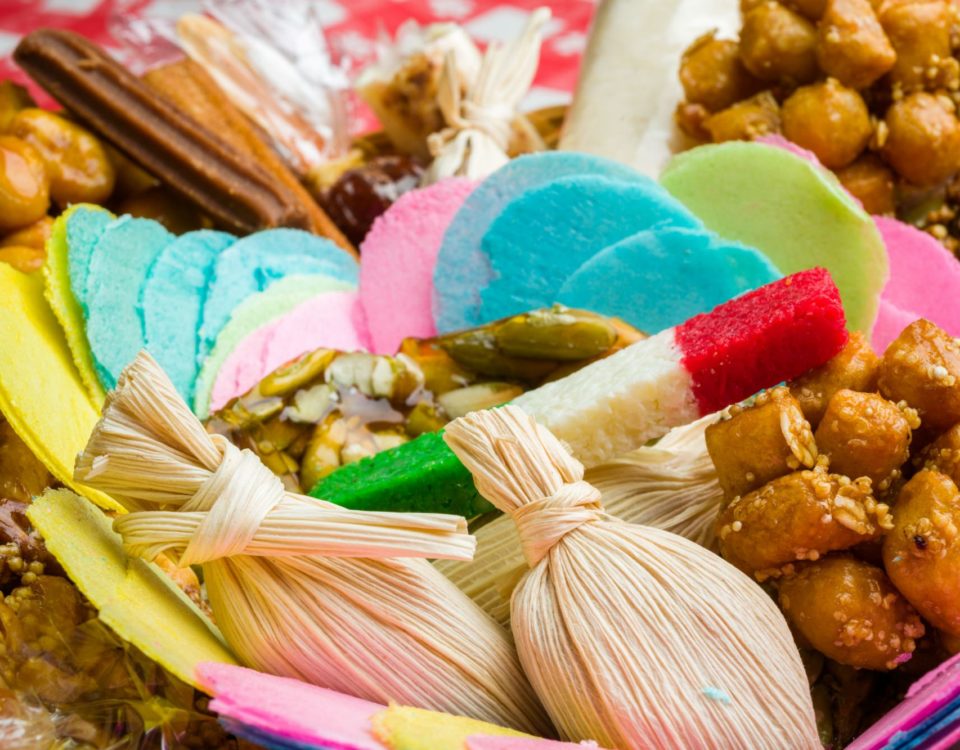This vibrant color photograph captures a delightful assortment of homemade-style confectioneries and treats, prominently featuring what appears to be Mexican cuisine. In the foreground, there are two items wrapped in corn husks, potentially tamales. Beside them, there are brown nuggets adorned with amber-colored sprinkles, possibly coated in sesame seeds. A striking item, a cube stick with a diagonal, green, white, and red striped pattern, suggests a festive Mexican treat. Central to the composition are wafer-thin colored discs in bright, eye-catching hues of teal, pink, light blue, and lime green. The background is filled with additional tamales and various colorful desserts, all arranged on a vibrant red cloth, enhancing the festive and appetizing appeal of the image.